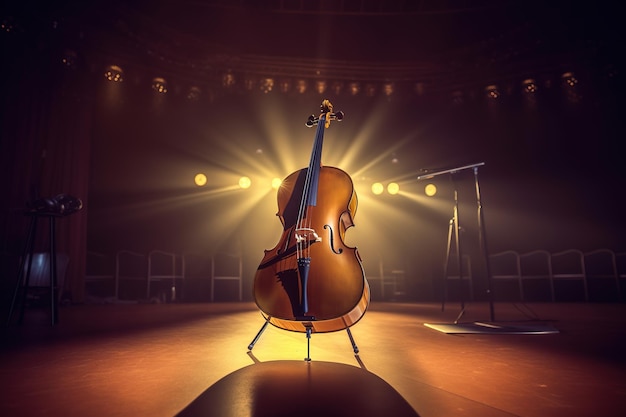This is a horizontally aligned, computer-generated stage image featuring a central brown cello standing upright on a tripod-like stand, which sits on a shiny brown floor. The cello's black neck and strings are clearly visible. To the right of the cello, there are several microphone stands with square bases and black poles, which are partially obscured and difficult to identify precisely. The background is illuminated by numerous yellow stage lights arranged in a horizontal line near the ceiling, casting rays of light that create a warm, golden-brown hue across the center of the stage and a shadow in the foreground. The top of the image reveals a dark ceiling adorned with gold decorations. Additionally, the stage features a red curtain at the back and some chairs are visible in the background, contributing to the realistic yet somewhat fantastical ambiance of the scene.